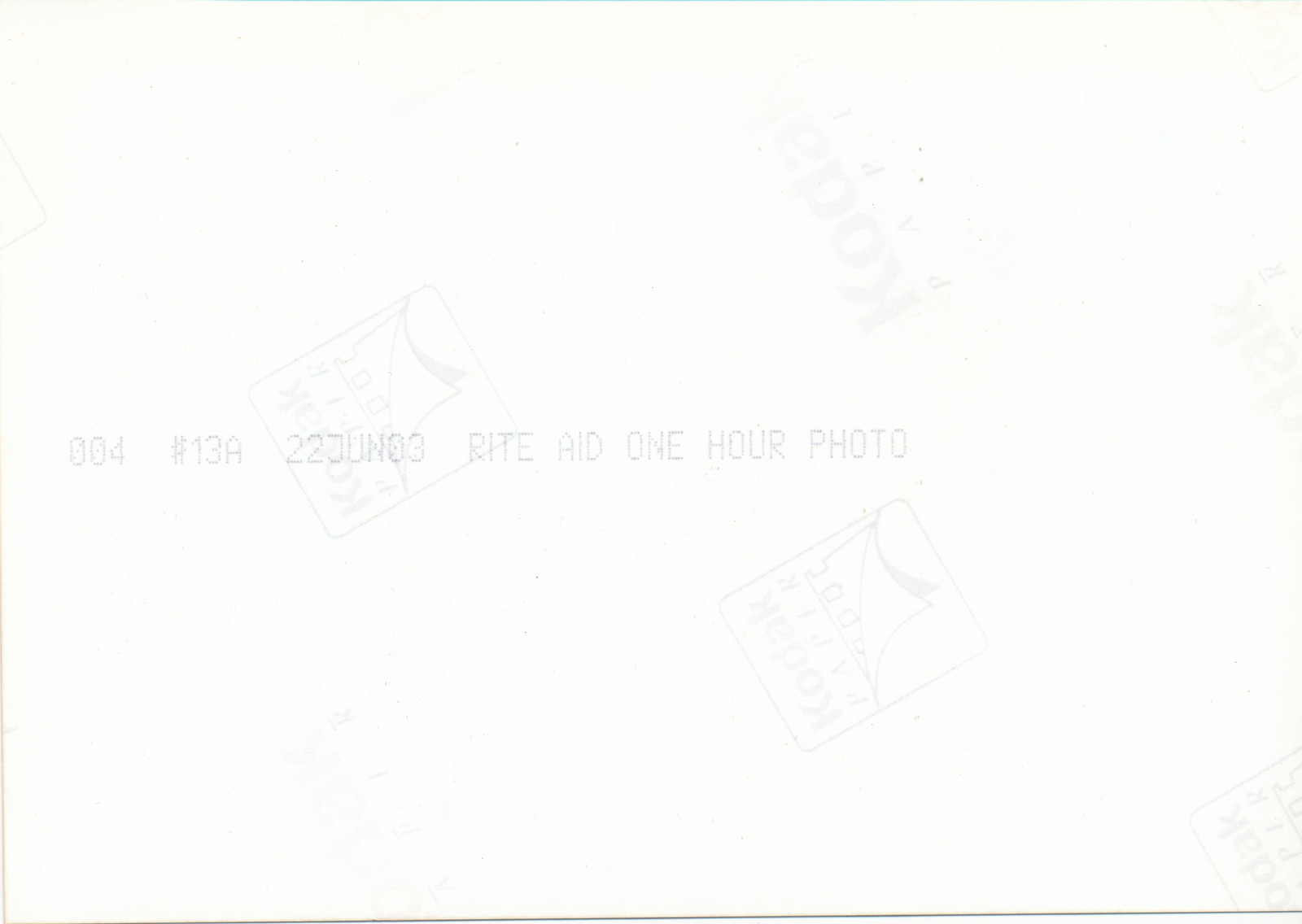A horizontally placed white rectangle dominates the image, resembling the back of a photograph. The only visible text is in capital letters and light blue font, reading "004  #13A  JUNO3  RITE AID  ONE HOUR PHOTO." Additionally, there are three extremely faint images on the back. One appears to spell out "KON," while the other two depict an image of a piece of paper being pulled away from another.